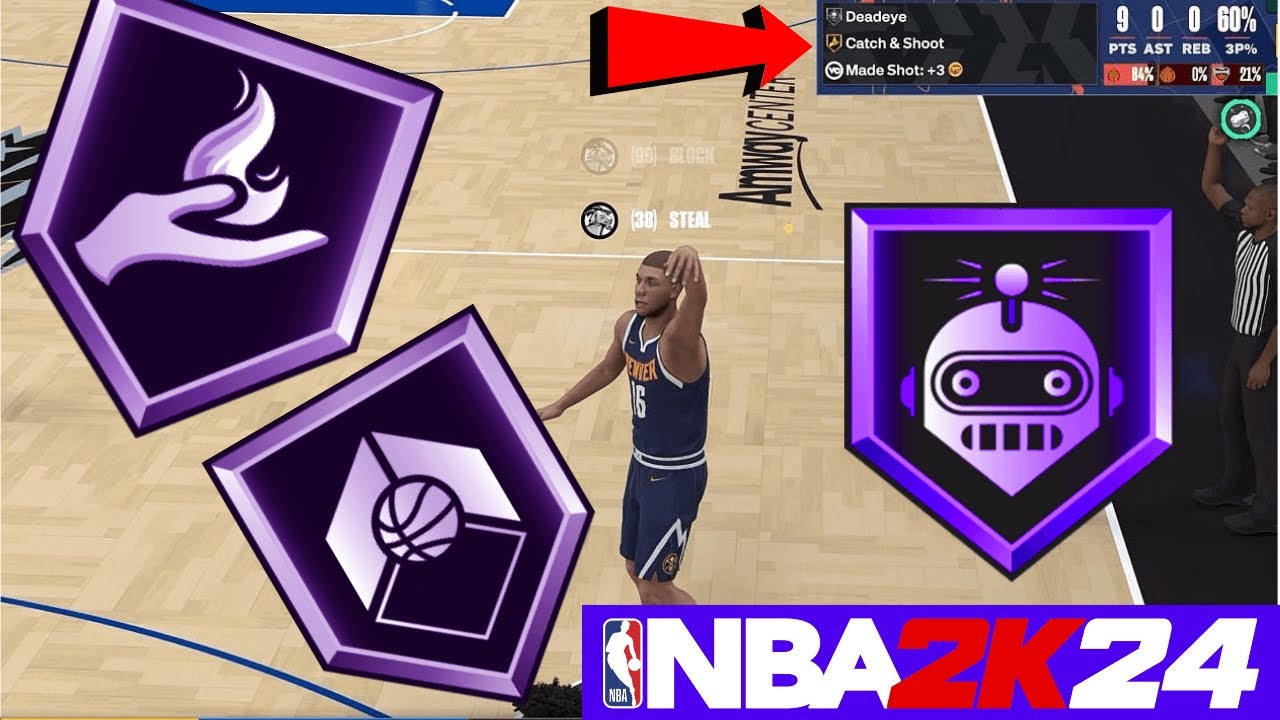A screenshot from the video game NBA 2K24 depicts an in-game basketball court, featuring a player wearing a navy blue jersey with white stripes and a yellow name emblazoned on the front. The player sports matching shorts, creating a cohesive athletic look. Off to the side of the court, a referee is standing with his hand raised; he's clad in the traditional black and white striped shirt.

In the upper right corner of the screen, a red arrow draws attention to a box that reads: "Dead Eye, Catch and Shoot, Made Shot, +3, 9 points, 0 assists, 0 rebounds, 60%". Surrounding this box are pentagon shapes with distinct designs on a purple background. The top-left pentagon depicts a hand with flames coming out of it, while the one beneath it features a design incorporating a basketball. The pentagon on the right shows a robot-like figure. At the bottom of the screen, adjacent to the NBA logo, is the game title "NBA 2K24".